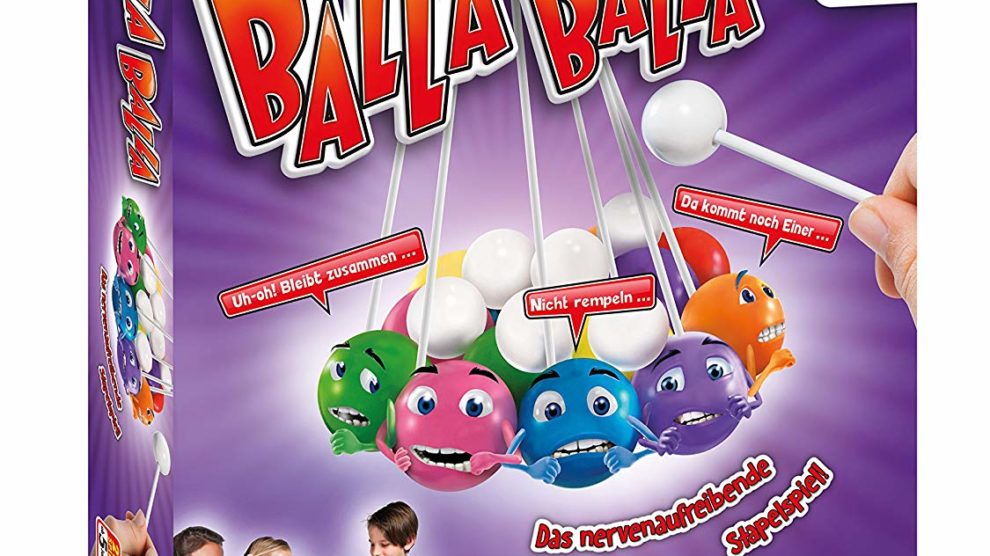The image portrays a vibrant, animated box for a child's game, predominantly enveloped in a radiant purple background that transitions to white in the center, radiating outwards. The top of the box showcases the bold red text "BALA BALA" with white borders. At the bottom, similarly styled red text reads "DAS NEVER NA FREBENDE STOPPEL SPIEL." Central to the image is a lively grouping of colorful spheres, in hues of green, pink, blue, yellow, purple, and orange, some adorned with faces, arms, and eyebrows, attached to strings. Above them, a layer of white balls seemingly rests atop the colored ones. A white stick with a spherical tip, held by a human hand emerging from the right side, appears poised to tap the balls. Red speech bubbles containing white text in an unreadable foreign language emanate from some of the spheres. In the lower left corner, the tops of three or four children's heads are slightly visible, adding a sense of playfulness and engagement to the scene.